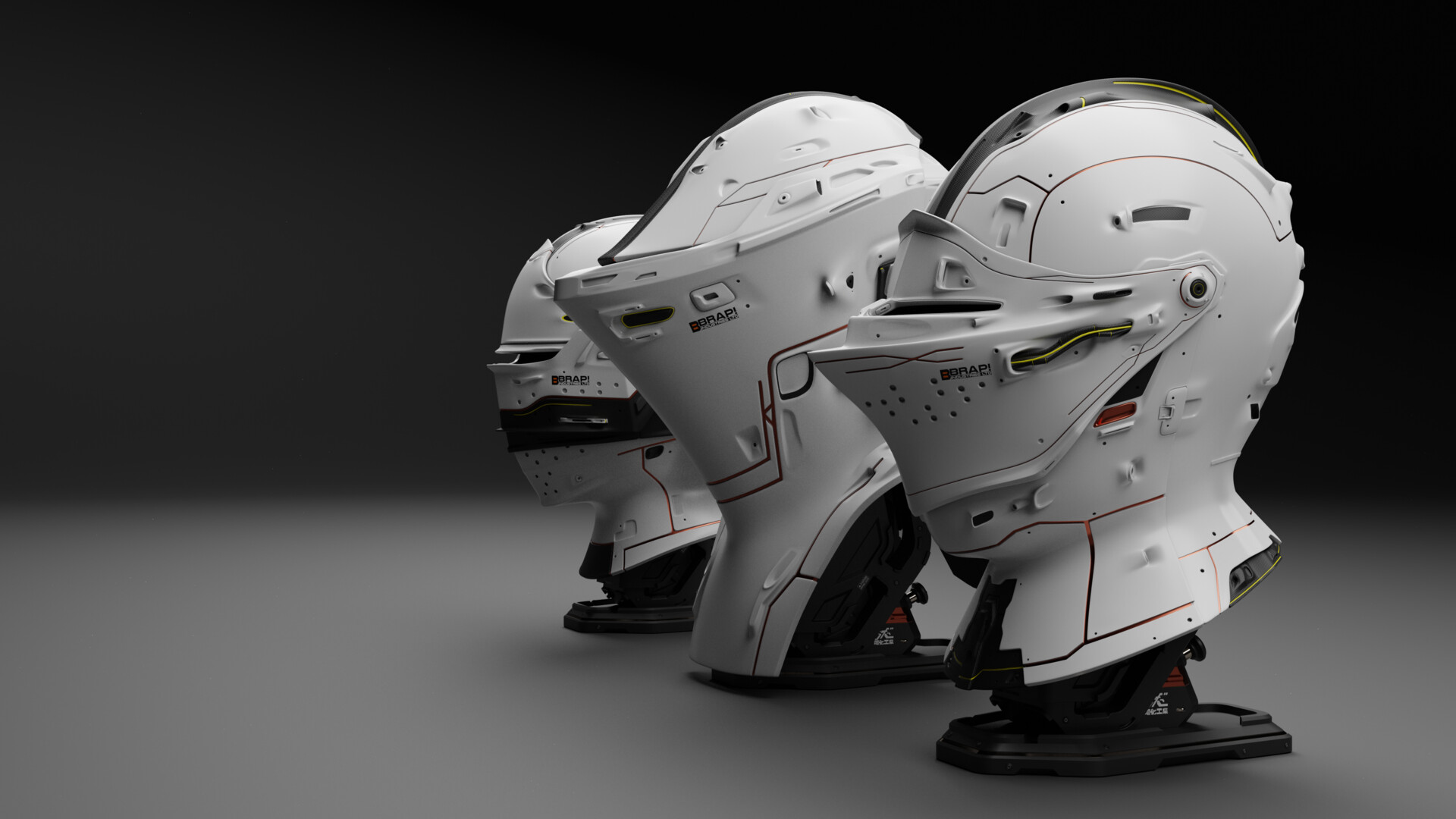The image showcases three futuristic, robotic-looking helmets, each predominantly white with varying designs and features. Positioned in a row, these helmets are displayed on black bases that obscure their actual scale, making it unclear whether they are human-sized or smaller pods. The closest helmet on the left combines elements from the other two: it has a rounded top and a front protrusion, possibly featuring a movable piece across the eyes. The middle helmet stands out with a mohawk-like ridge in its plastic, emphasizing its unique shape. The farthest helmet is more rounded and appears smallest, with distinct slits indicating potential eye placement and a noticeable black band beneath. All helmets share a sci-fi aesthetic reminiscent of something from a Star Wars movie and have the label "be prep!" with an exclamation mark.